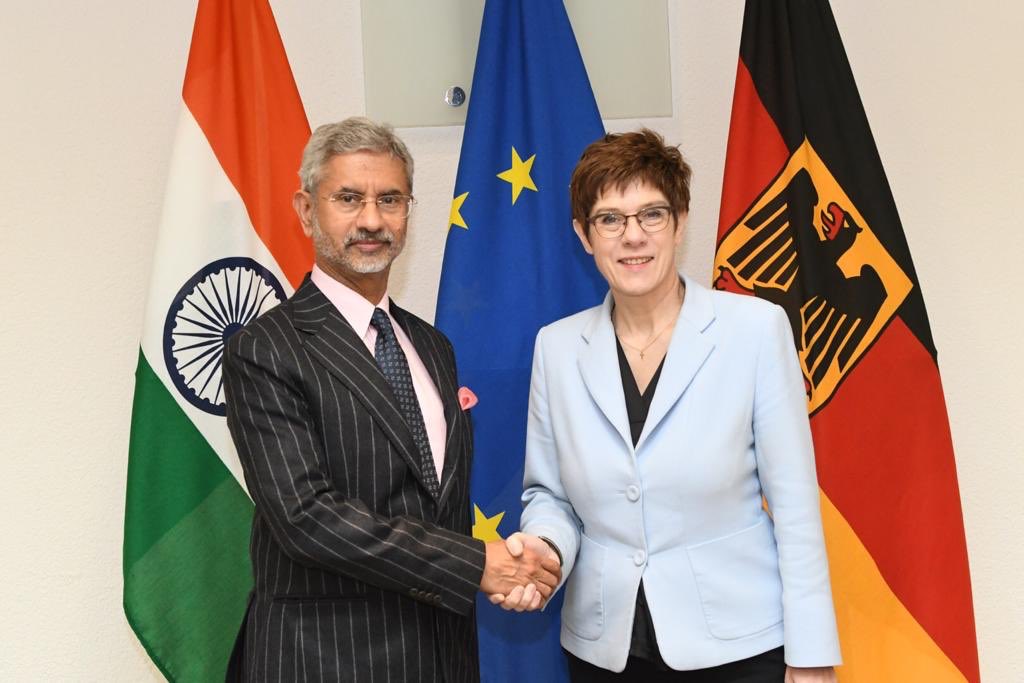In the image, a man and a woman are standing side by side in front of a white wall adorned with three distinct flags. Both individuals are looking directly into the camera while shaking hands. The man, positioned to the left, is dressed in a navy blue and light blue pinstripe suit, complemented by a pink shirt and a matching navy and light blue tie. He has gray hair, a neatly trimmed gray beard and mustache, and he is wearing glasses. The woman, slightly younger and standing to the right, sports a navy dress paired with a light blue jacket and a gold necklace. Her red hair is styled in a pixie cut, and she also wears glasses.

Behind them, the leftmost flag features green, white, and red vertical stripes, indicative of Italy. The central flag is blue with yellow stars, possibly representing the European Union. The rightmost flag is striped black, red, and yellow, showcasing an imposing bird emblem, resembling the German flag. The setting suggests a formal international event, potentially an economic summit or diplomatic meeting, characterized by a brightly lit room.